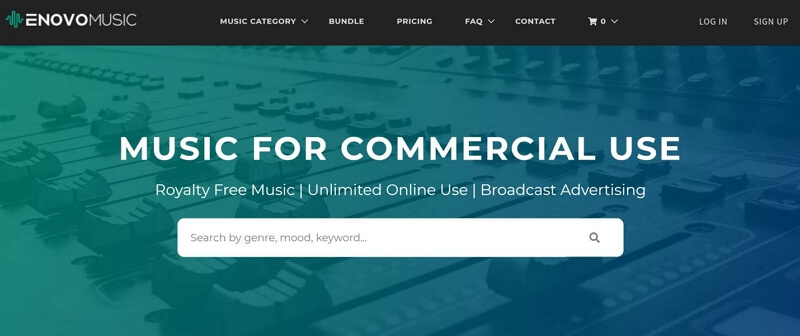The image depicts a screenshot of a webpage for N. Ovo Music. At the top, a black banner with white text displays the site name "N. Ovo Music" alongside a green logo. Below the banner are various navigational options in white text: "Music Category" with a drop-down menu, "Bundle", "Pricing", "FAQ" with a drop-down menu, and "Contact". On the right side of the banner, there are icons for a shopping cart with a drop-down, login, and signup options.

Dominating the center of the page, large, bold text reads "Music for Commercial Use" with a background featuring musical studio equipment such as slider bars and buttons. Beneath this, smaller white text states "Royalty Free Music", "Unlimited Online Use", and "Broadcast Advertising". Also near the center is a white search bar with a magnifying glass icon and placeholder text saying "Search by genre, mood, and keyword".